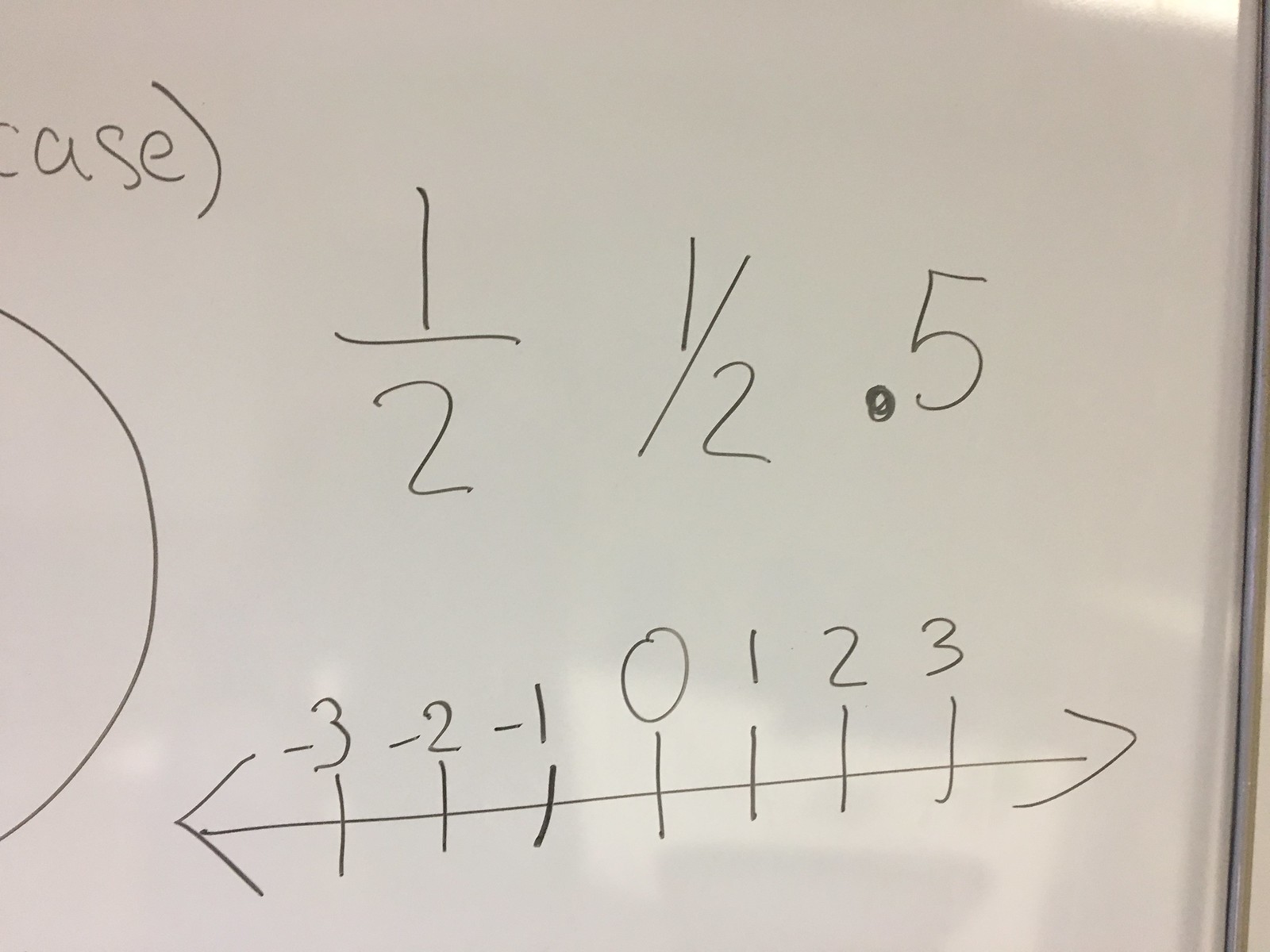This color photograph features a white dry-erase board with various markings and writings, reflecting some ambient light without clear visible reflections. On the far left of the image is the word "CASE" followed by a closed parenthesis. A semicircle stretches from the approximately left center of the board down to just above the bottom left corner. In the middle section of the board, there are symbols and numbers: "1" with a vertical line, "2", "1" with a diagonal line, "2", and "point 5."

At the bottom of the board is a double-ended arrow, with one arrowhead pointing to the left and the other to the right, connected by a long horizontal line. Along this line are numerous thin vertical tick marks. Above these tick marks are the numbers labeled from left to right as "-3, -2, -1, 0, 1, 2, 3." On the far right edge of the photograph, a small portion of the metallic frame of the whiteboard is visible.